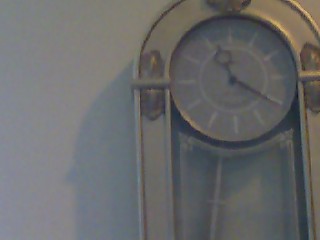The image depicts a slightly blurry, color photograph of an analog clock mounted on a light grey, possibly pearl grey, wall. The clock, situated on the right side of the photograph, features a distinctive U-shaped frame facing down, with a combination of grey and brown colors, and has silver clasps on the sides and top. Inside the clock, the face is grey with white dashes instead of numbers to indicate the hours. The black hour hand points just past 11 while the black minute hand points to the 4, indicating the time is approximately 11:20. There is a pendulum or similar swinging part at the bottom of the clock, currently swinging towards the left. The overall lighting in the photograph is dim, contributing to the muted color tones, and a shadow is visible on the wall to the left of the clock.